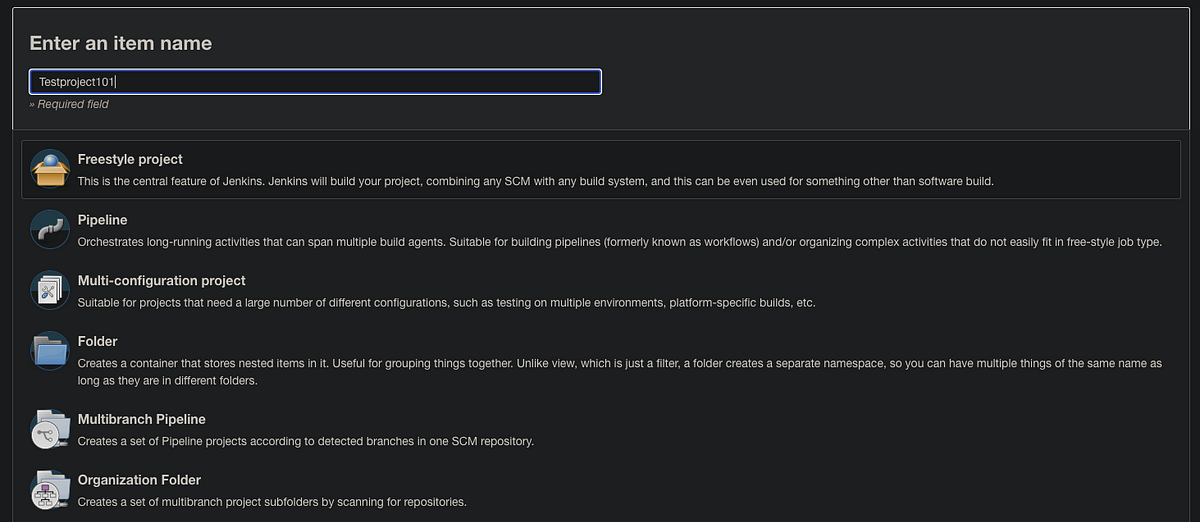The image depicts a website interface with a minimalist, black background. At the top, in white text, it prompts the user to "Enter an item name." Directly below this field, it displays "Test Project 101," with an adjacent note stating "Required field."

Continuing downward, the interface lists several project types, each accompanied by a brief description in white text. The options include:

1. **Freestyle Project**: This is a central feature of Jenkins.
2. **Pipeline**: Orchestrates long-running activities that can span multiple build agents.
3. **Multi-Configuration Project**: Suitable for projects that require a large number of different configurations.
4. **Folder**: Creates a container that stores nested items in it.
5. **Multi-Branch Pipeline**: Creates a set of pipeline projects based on detected branches in a single SCM repository.
6. **Organization Folder**: Generates subfolders for multi-branch projects by scanning repositories.

At the bottom of the page, there appears to be a screenshot showing a section of a software image, presumably captured from the user's computer. The detailed descriptions clearly outline the functionalities of each project type, taking advantage of the high contrast between the black background and white text for clarity.